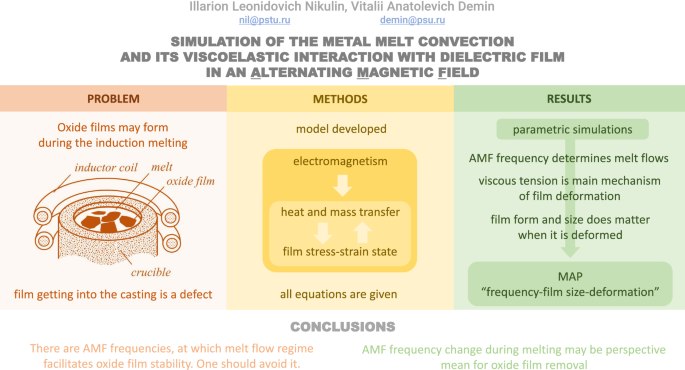The image is a detailed technical infographic illustrating the simulation of metal melt convection and its viscoelastic interaction with dielectric film in an alternating magnetic field. It is structured in a three-part, color-coded diagram against a white background, with labeled sections for Problem (on a light red background), Methods (on a yellow background), and Results (on a green background). 

Starting from the left, the "Problem" section indicates that oxide films can form during induction melting, which is shown with a diagram of a crucible containing melting metal and an oxide film within an inductor coil. The text explains that the inclusion of this film into the casting process is considered a defect.

The center "Methods" section explains the developed model focusing on electromagnetism, heat and mass transfer, and the ensuing film stress and strain states. This section is detailed with equations that underpin the model's framework.

The "Results" section on the right demonstrates parametric simulations showing that the alternating magnetic field (AMF) frequency determines melt flows, with viscous tension identified as the primary mechanism of film deformation. It emphasizes the significance of film form and size during deformation. The conclusion, noted at the bottom, highlights that specific AMF frequencies promote oxide film stability, which should be avoided, suggesting that changing the AMF frequency during melting could be an effective means for oxide film removal.